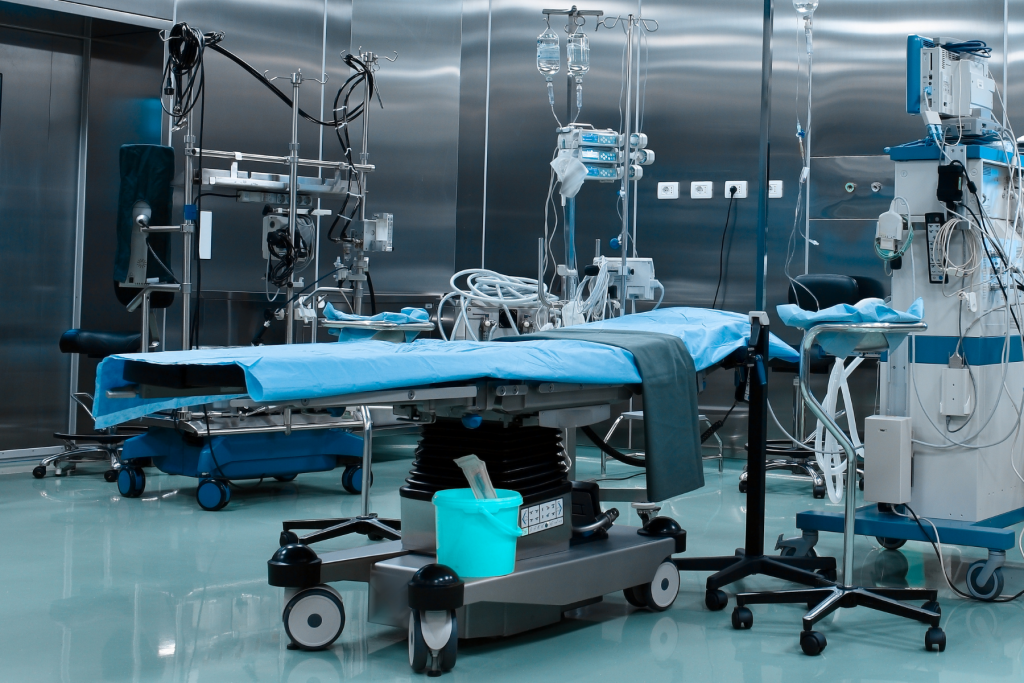The photograph captures an unoccupied, meticulously clean operating room inside a hospital. Dominating the center is an electrical gurney, draped in a blue medical sheet, topped with a smaller gray sheet. Below the gurney, on its wheeled platform, lies a teal-colored bucket. To the right of the gurney stands a piece of medical equipment, likely for monitoring vital signs, identifiable by its screen and numerous cords protruding from the back and sides. Nestled between this device and the gurney, a mobile instrument tray with a blue medical sheet tucked inside awaits use. The background reveals an assortment of hanging IVs and additional medical apparatus, all set against metallic, stainless steel walls that gleam under the room's lighting. The expansive floor, made of shiny, ceramic-like tiles, accentuates the room’s sterile and orderly environment. An open doorway is visible to the far left, hinting at the vast network of corridors beyond.